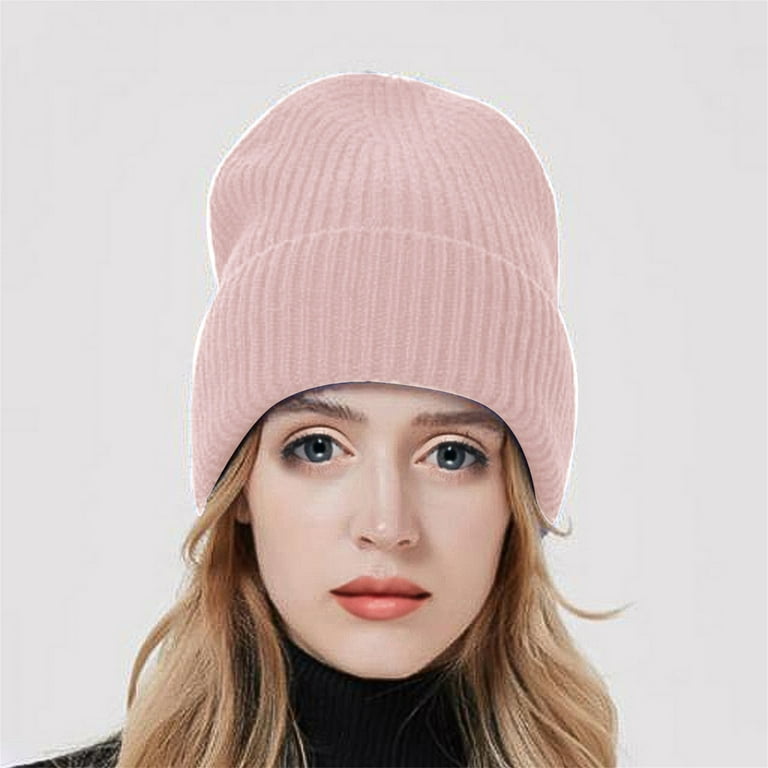The image depicts a close-up of a young woman with a light complexion, gazing directly into the camera. She is wearing a light pink, knitted beanie that is tall and rolled-up just above her forehead, allowing her light brown to blonde hair to flow down to her shoulders. The woman’s eyes are a bluish-gray color, complemented by well-groomed brunette eyebrows. Her lips are painted a peachy red hue. She has on a black turtleneck sweater, and the photograph cuts off just below her shoulders. The background is stark white, and the image overall is a bit blurry and low in resolution, although the lighting ensures the subject is brightly and clearly seen.